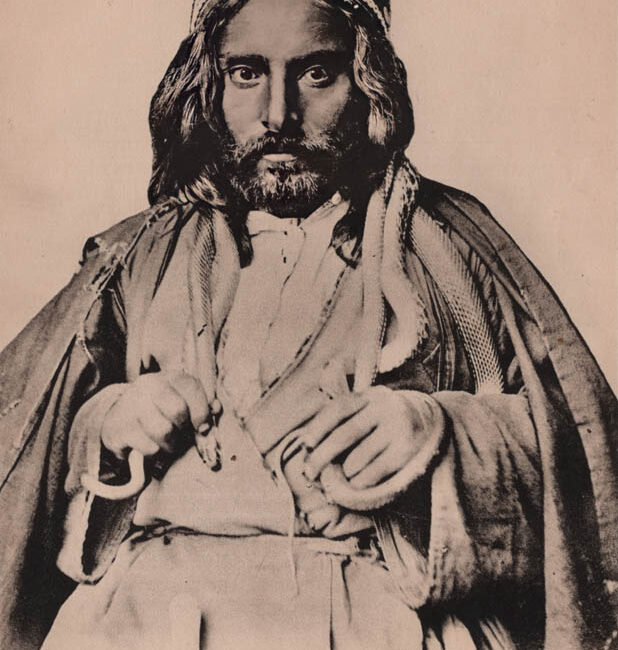This detailed black and white photograph, enhanced with a sepia tone, features a man with long, stringy hair, a salt-and-pepper beard, and dark skin. His attire includes several layers of robes, and he is wearing a hat on his head. Around his neck and draped over his hands are multiple snakes, which he grips cautiously, possibly to prevent them from biting. The snakes, which could be mistaken for thin, noodle-like objects at first glance, blend into his hair and add to the overall enigmatic atmosphere of the image. The sepia tone gives the photograph an old, foreign feel, reminiscent of an ancient or historical portrait. It evokes a sense of mystique, with the man’s appearance and attire suggesting a possible cultural or ethnic significance, given the combined descriptions suggesting anything from a Hebrew figure to a character like Jack Sparrow from Pirates of the Caribbean.